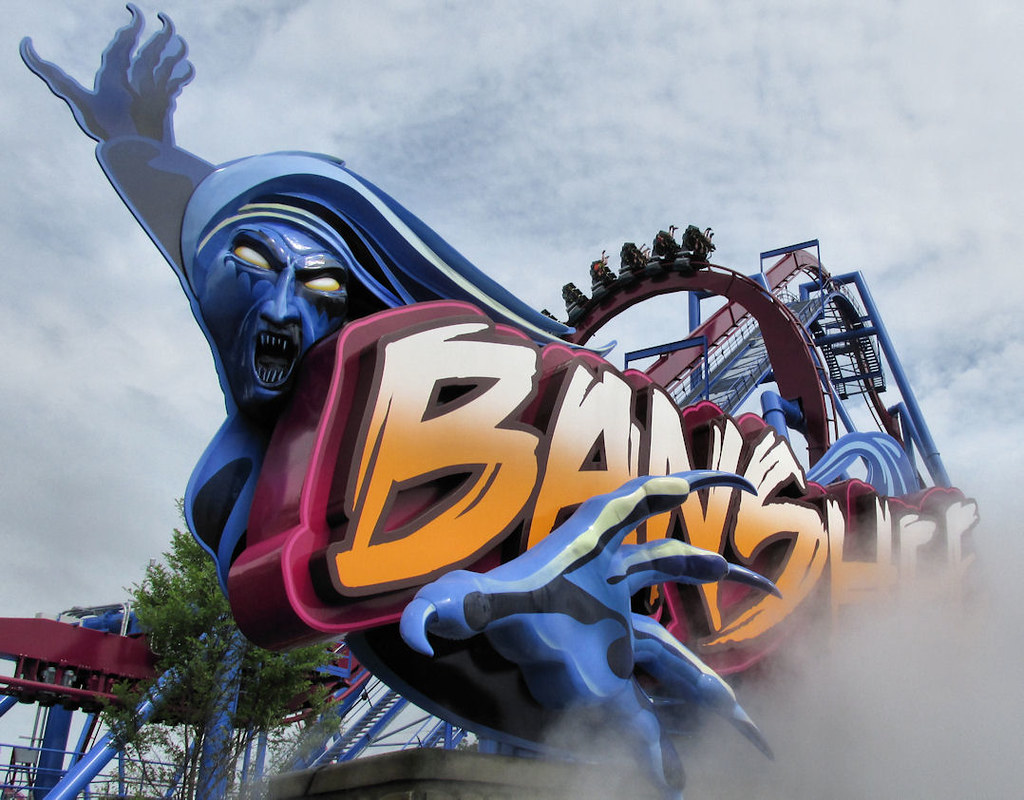The image captures a vibrant and detailed scene at an amusement park featuring the "Banshee" roller coaster. Dominating the view is a striking logo with an orange and white design, featuring a large banshee figure with long hair, ghoul-like purple eyes, and sharp, razor-like teeth. This banshee character is depicted in vivid blue with menacing claws stretching outwards; one hand reaches skyward while the other extends menacingly forward.

The roller coaster itself is a striking combination of purple, blue, and burgundy, with a large metal frame and visible tracks that loop up and down. Riders are strapped in, hands raised in anticipation as they prepare to descend from a high peak. In the lower sections of the image, a tree stands at ground level, adding a touch of nature to the scene. The sky above is predominantly blue with patches of cloud cover.

Additional visual elements include the fog or smoke partially obscuring the bottom right corner, accentuating the eerie and thrilling atmosphere. In the background, another section of the ride is visible, providing a glimpse of the ride's extensive, looping structure. This carefully constructed image captures the energy, anticipation, and detailed design of the "Banshee" roller coaster, set against a dynamic daytime sky.